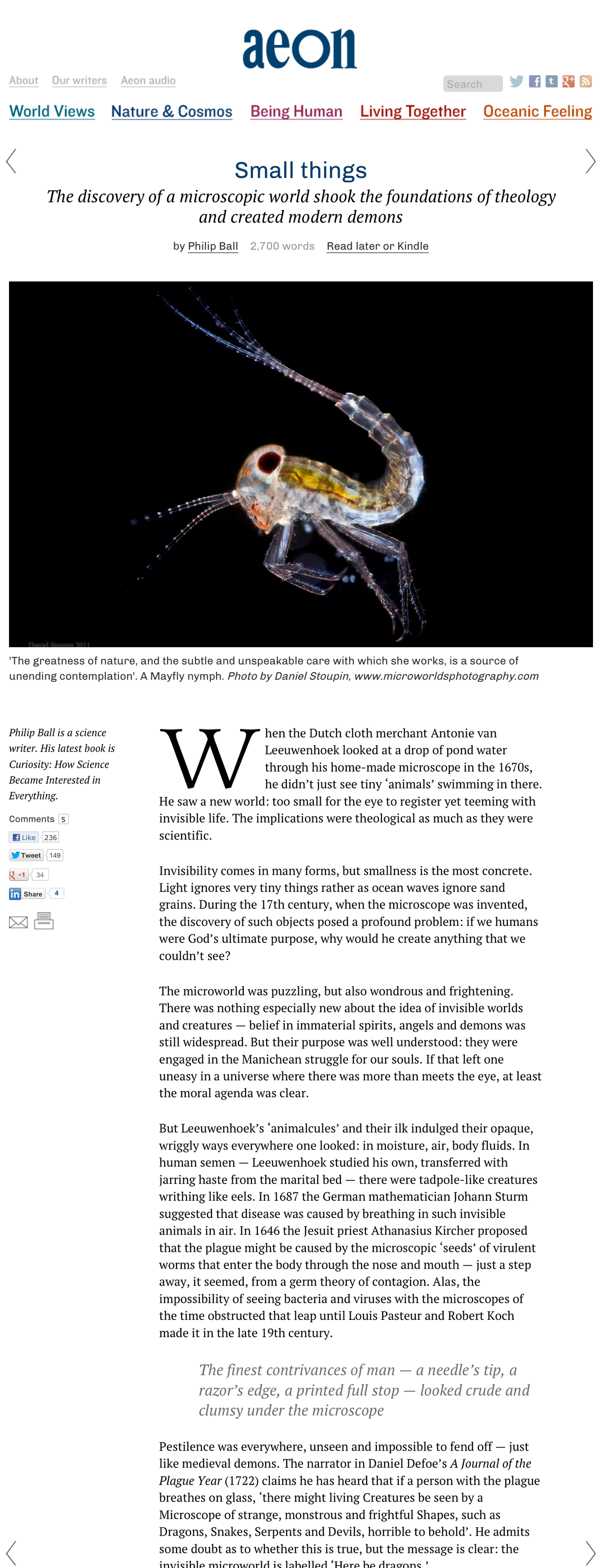This is a screenshot of the Aon website, which features a predominantly white background and extensive text. The site appears to deliver news on various biological and natural science topics, categorized under themes such as Worldviews, Nature and Cosmos, Being Human, Living Together, and Oceanic Feeling. The highlighted news article is titled "Small Things: The Discovery of the Microscopic World Shook the Foundations of Theology and Created Modern Demons." 

An image of an unidentified sea creature, possibly a shrimp, accompanies the article. The image's backdrop is black, providing a stark contrast that highlights the creature's details. The caption under the image reads, "The greatness of nature and the subtle unspeakable care with which she works is a source of unending contemplation."

To the left of the article, there is a brief author's bio, stating that Philip Ball, a science writer, authored a book titled "Curiosity: How Science Became Interested in Everything." Additionally, the website includes interactive icons for comments, social media likes, email sharing, and printing.